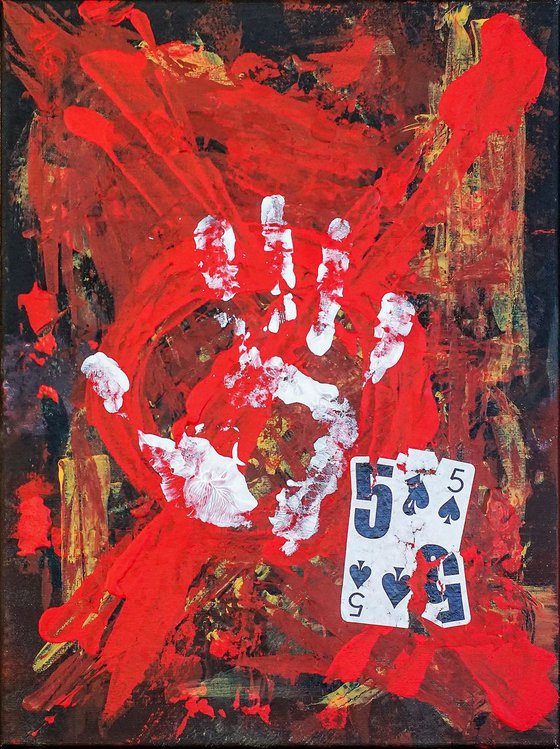This abstract painting is a striking modern art piece, prominently featuring a white handprint at its center, with the thumb oriented to the left and the fingers reaching upwards. The rectangular canvas is painted with a dark background, layered with bold, vivid strokes of red and yellow. A distinct red "X" stretches diagonally across the canvas, intersected by an encompassing red circle. Thick yellow lines add to the textured complexity of the composition. 

In the lower right-hand corner, there is a prominently featured, pieced-together playing card, the Five of Spades, which is torn and reassembled like a puzzle. The number five on the card is exaggerated, appearing significantly larger in the upper left and bottom right corners compared to the other corners. The artwork's design and color scheme evoke a sense of intensity and dynamism, with varying brush strokes and paint splashes adding to its textured appeal.